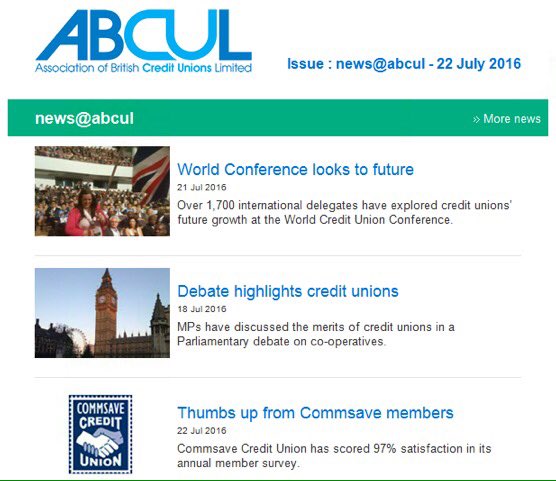### Newsletter from the Association of British Credit Unions Limited (ABCUL) - July 22nd, 2016

#### Top Header Section
- **Logo**: Positioned in the upper left-hand corner, the ABCUL logo features the letters "A" and "B" capitalized in navy blue, while the "C" and "U" are in a lighter shade, emphasizing the union of British Credit Unions. The "L" returns to navy blue, highlighting the Limited aspect of the organization's name.

#### Main Article
- **Headline**: Over 1,700 International Delegates Attend Conference
  - **Content**: The newsletter's main article details a significant conference attended by more than 1,700 international delegates. The focus of the conference was exploring the future growth and development of credit unions worldwide.
  - **Image**: Accompanying the article is an image showing a large crowd, presumably taken at the conference, capturing the event's extensive participation and dynamic atmosphere.

#### Secondary Articles
- **Debate Highlights in Credit Unions**
  - **Content**: A secondary piece discussing critical debates on pivotal issues affecting credit unions, reflecting diverse perspectives and highlighting significant discussions from the event.

- **Thumbs Up from Palm Save Members**
  - **Content**: This section features a positive response from Palm Save members, depicted through an image of shaking hands with the credit union emblem, symbolizing mutual support and collaboration within the credit union community.

#### Visual Elements
- Multiple images enhance the storytelling, including a large crowd at the conference and symbolic gestures of cooperation and approval among credit union members.

This detailed newsletter provides comprehensive coverage of key events and discussions relevant to the credit union industry, highlighting ABCUL's role in fostering international dialogue and collaboration.